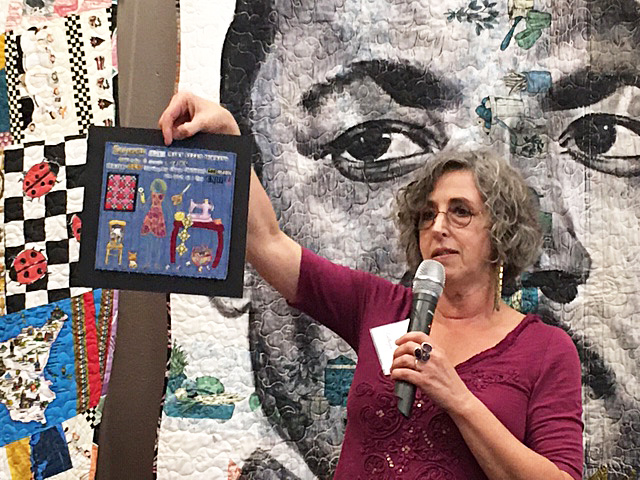An older white woman in her 60s with curly, chin-length gray hair and glasses stands in the forefront of the image, holding a microphone in her left hand. She wears dangling gold earrings, a maroon short-sleeved blouse adorned with sequins and embroidered designs, maroon lipstick, and rings on her fingers. Her right hand holds up a framed illustration with a blue background, depicting a scene with a chair, a dress, a table, and a sewing machine. Behind her, a mural of Martin Luther King Jr. in black and white dominates the background, with blue and green foliage details. To the left, a colorful quilt featuring ladybugs and various abstract designs is visible. The scene suggests an event focused on art or history, with quilts and illustrations prominently displayed around her.